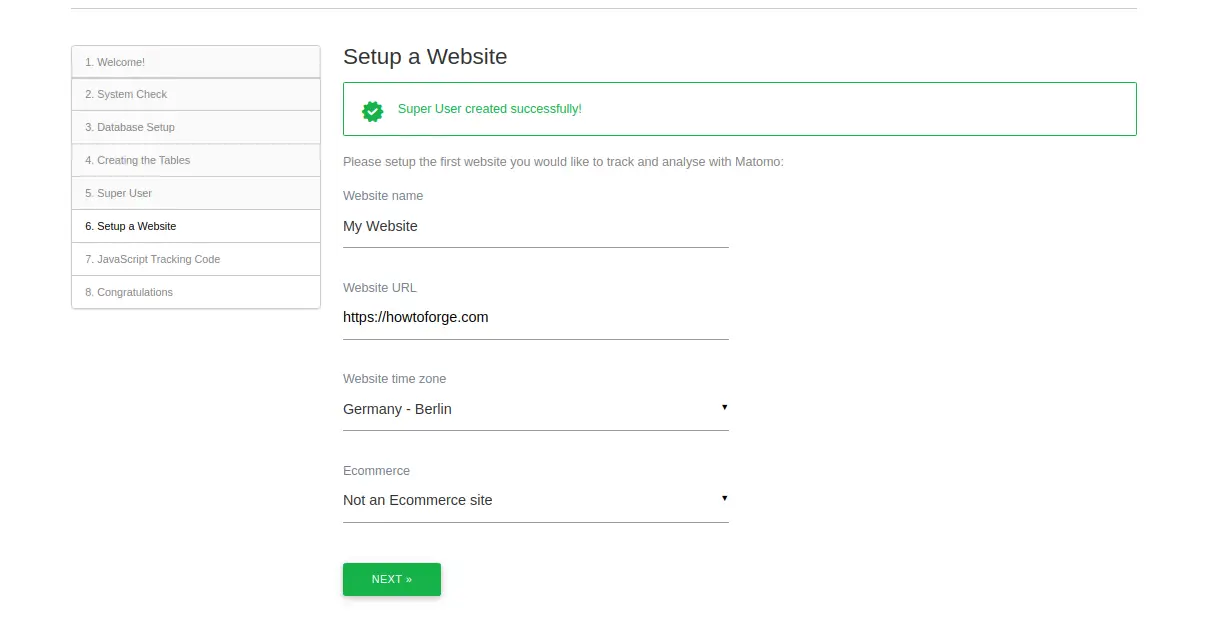Screenshot of Matomo Setup Wizard: Detailed Section Breakdown

The screenshot is divided into two sections: a sidebar on the left and the main content on the right.

**Left Sidebar:**
- It's a step-by-step navigation chart with eight lines indicating the setup progress:
  1. Welcome
  2. System Check
  3. Database Setup
  4. Creating the Tables
  5. Super User
  6. Set Up a Website (this step is highlighted)
  7. JavaScript Tracking Code
  8. Congratulations

**Main Content Area:**
1. **Title:** The main title displayed prominently is "Set up a website."
2. **Success Message:** Below the title, there is a green box with a green outline and a green check mark, containing the text "Super User created successfully."
3. **Instruction:** Following the success message, there is a line with smaller text that reads: "Please set up the first website you would like to track and analyze with Matomo."
4. **Form Fields:**
   - **Website Name:** A labeled line for entering the website name.
   - **Website URL:** A labeled line for entering the website URL, with an example provided as "howtoforge.com."
   - **Website Time Zone:** The selected time zone is "Germany, Berlin."
   - **E-commerce:** The selected option indicates that the site is "Not an e-commerce site."
5. **Next Button:** At the bottom of the form, there is a green "Next" button for proceeding to the next setup step.